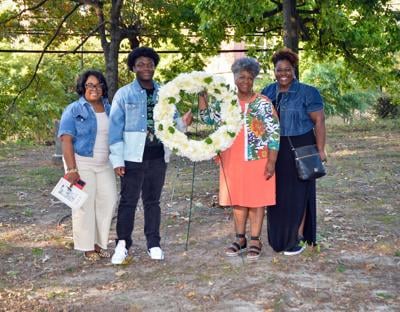The photograph depicts a group of four African-American individuals standing outdoors in a casual setting, possibly during the spring or summer. They are arranged around a stand holding up a white wreath adorned with green leaves. From left to right: there's a woman in a denim top, a young boy also in denim, a middle-aged woman in a floral top with an over sweater and sandals, and a woman in a long maxi dress with a denim jacket and cross-body purse.

The ground beneath them is light brown and gray, dotted with sparse patches of grass, sticks, and leaves. In the background, a line of lush green trees and bushes can be seen, along with some power lines running across the scene. Despite being outdoors in a somewhat rough terrain, the group stands together with big smiles, suggesting a joyful moment.